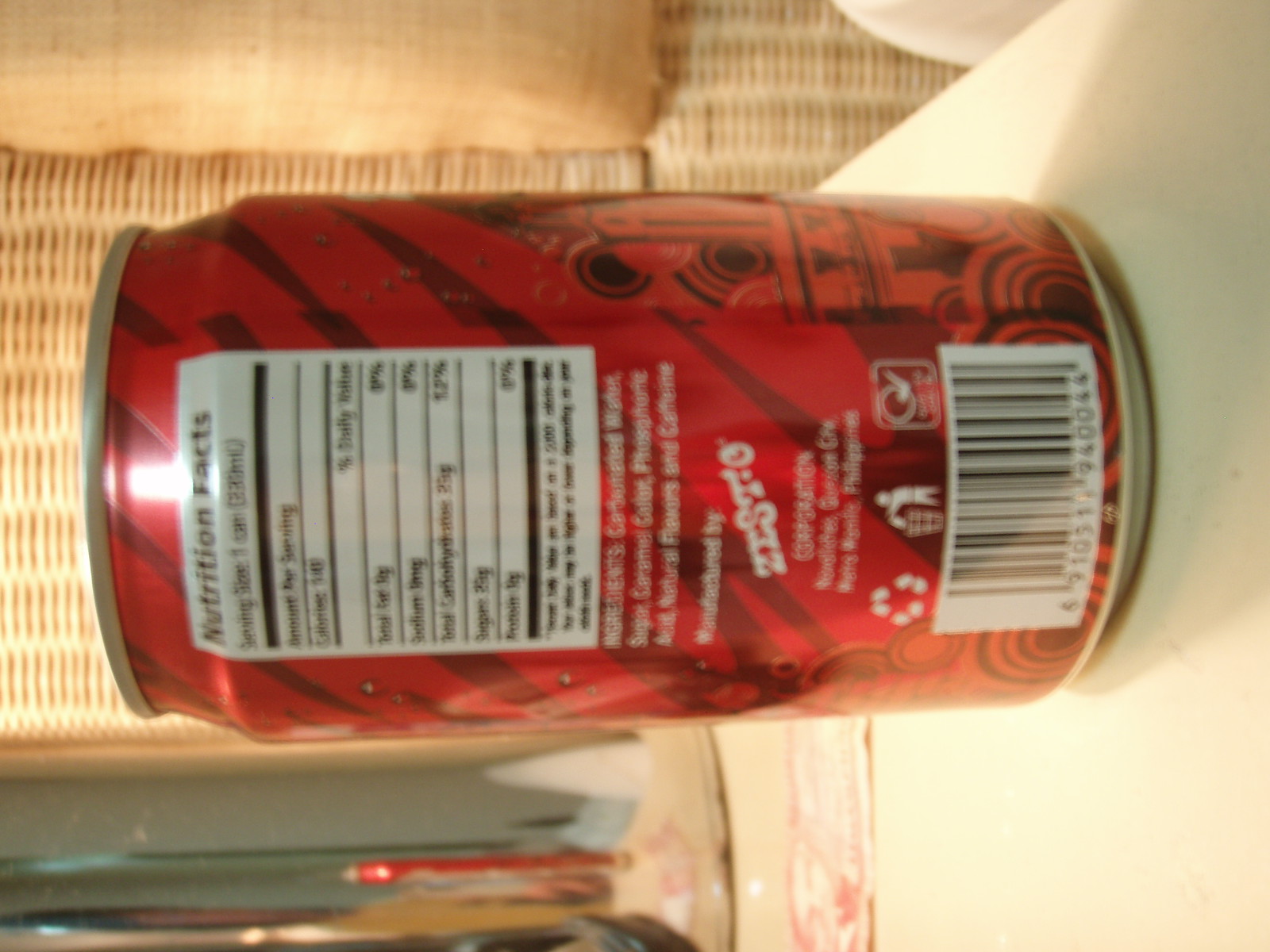This image depicts a red aluminum beverage can lying on its side, tilted to the left. The photograph is slightly out of focus, making finer details challenging to discern. The can features a red background adorned with black patterns, including stripes and concentric circles. Visible elements include a barcode, a white recycling symbol, and an icon of a person disposing of trash into a bin. The brand name appears to be "ZISTO," though the text is not entirely clear due to the blurriness of the image.